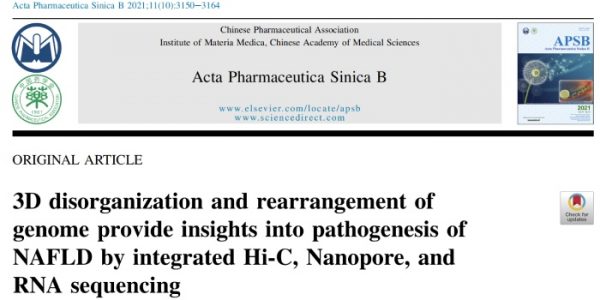Screenshot of a website featuring the header of a scientific journal publication. The background is predominantly white, with the journal's title displayed in a greenish-blue font: "Acta Pharmaceutical Seneca B 2021: 11(10): 3150-3164." Below the title is a banner with a gray center flanked by white on either side. On the left side of the banner, there are two circular icons stacked vertically. The upper icon is navy blue and features an open book symbol, while the lower icon is red with Chinese characters around a central Chinese symbol.

Occupying the center of the banner is a gray rectangle with black text that reads: "Chinese Pharmaceutical Association Institute of Materia Medica Chinese Academy of Medical Science Acta Pharmaceutical Seneca B." Below this text are two website links: "www.elsevier.com/locate/APSB" and "www.sciencedirect.com," providing additional resources and access to the journal's contents.